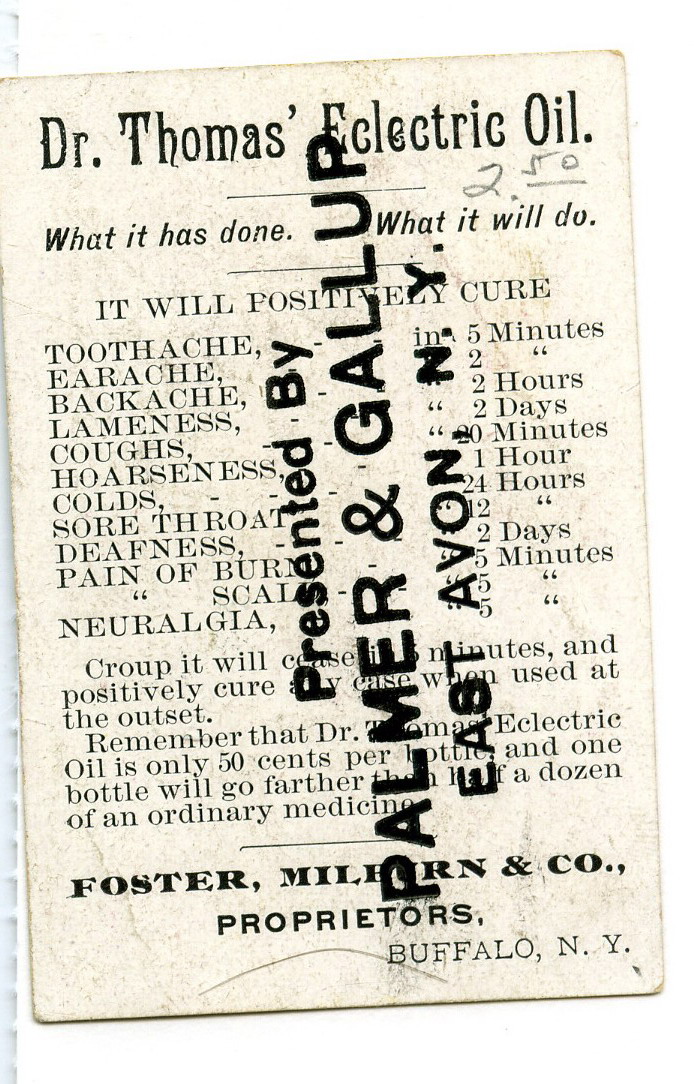The image is of a white card with black text, titled "Dr. Thomas's Eclectic Oil." The text details the various ailments the oil claims to cure, specifying durations for each: toothache in five minutes, earache and backache in two hours, lameness in two hours, coughs in 20 minutes, hoarseness in one hour, colds in 24 hours, sore throats in 12 hours, deafness in two days, pain from burns in five minutes, scalp issues in five minutes, and neuralgia in five minutes. However, some text is obscured by a stamp that reads "Presented by Palmer and Gallup, East Avon, New York." The card also mentions Foster, Milburn, and Company, proprietors based in Buffalo, New York. Additionally, someone has written "2.50" on the card, possibly indicating its price.